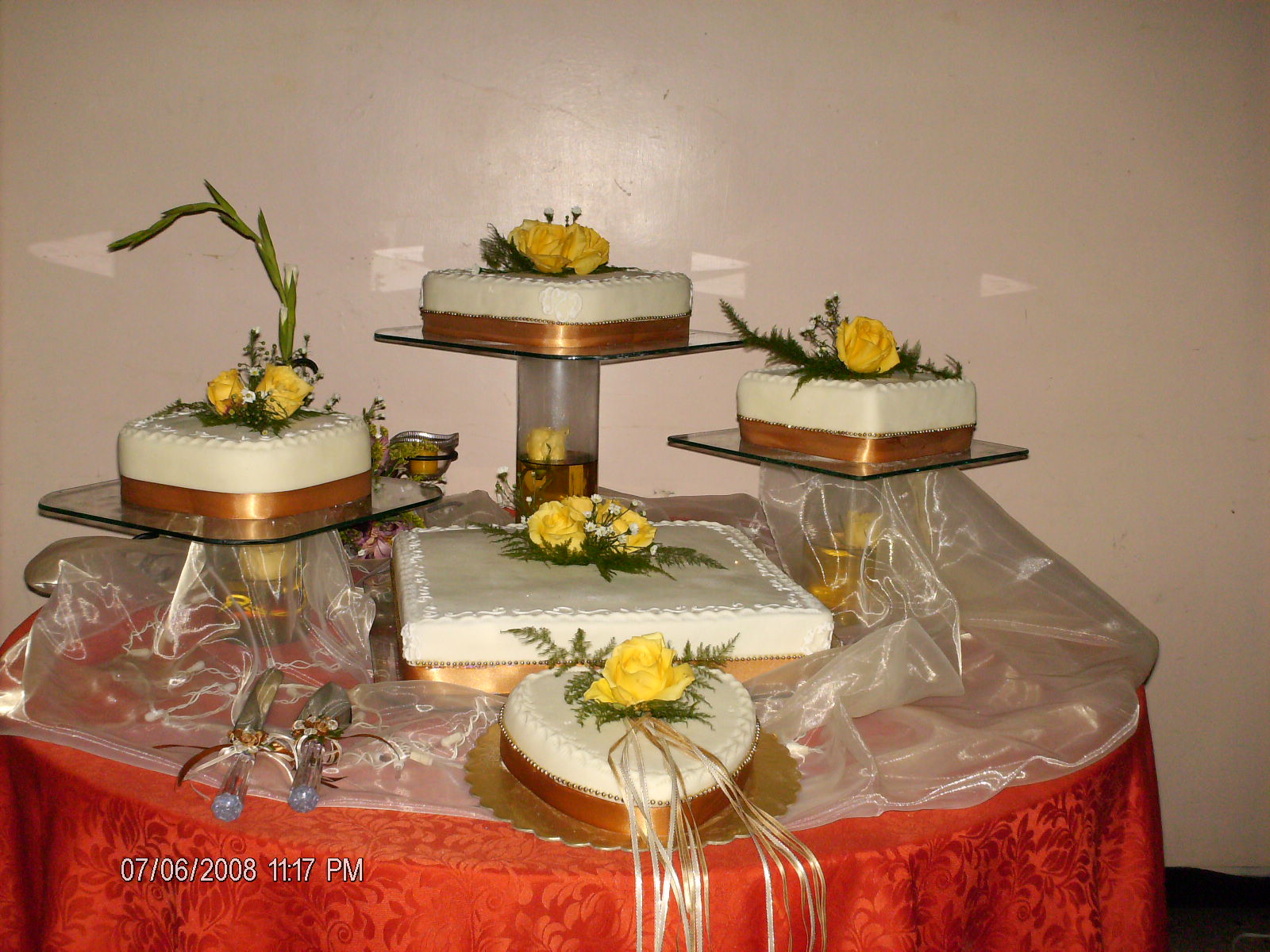This color photograph captures an intricately arranged indoor display of cakes on a large, round table draped with a striking red tablecloth. The setup features five distinct cakes, all adorned with white frosting and garnished with yellow roses at the center of each. The cakes vary in shape: one large rectangular cake, a heart-shaped cake positioned near it, and three additional heart-shaped cakes elevated on stands behind the rectangular cake. The display is further detailed with a knife and serving spoon placed to the left side. A time stamp in the bottom left-hand corner reads "July 6, 2008, 11:17 p.m." The backdrop to this tableau is a tan wall, contributing to the focus on the cakes, which resemble a wedding-style presentation.